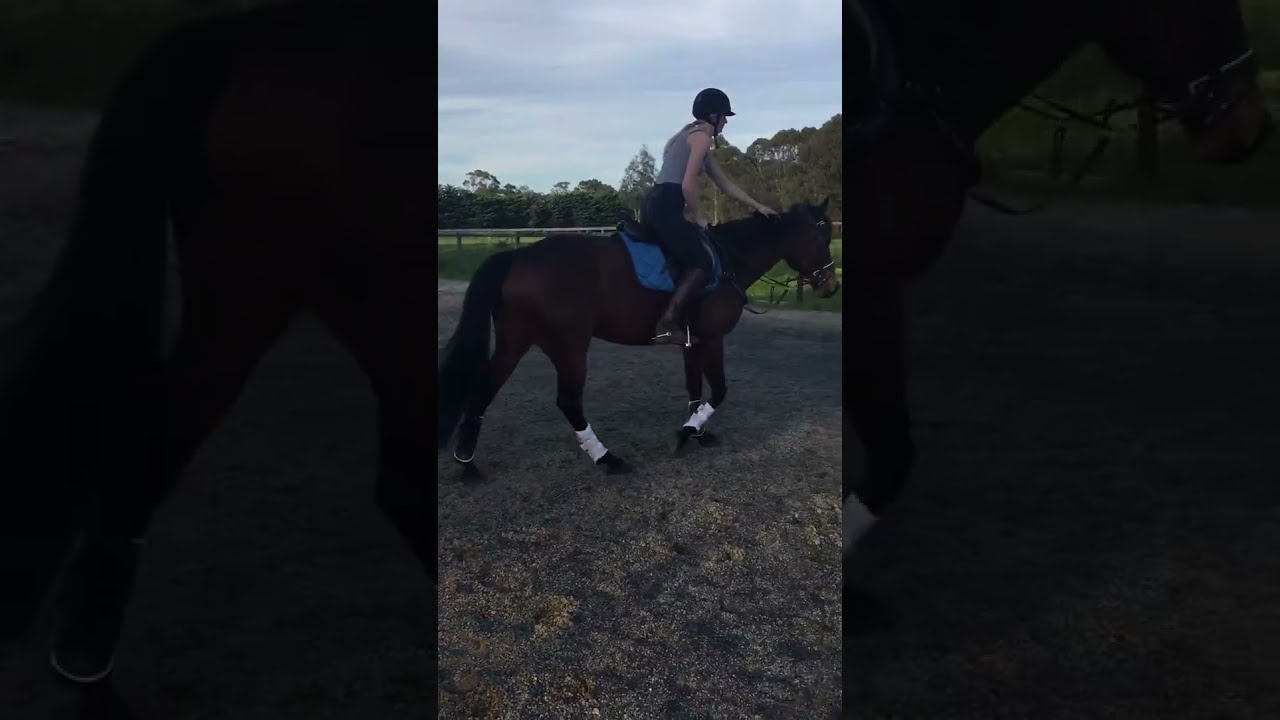A woman sits atop a dark brown thoroughbred horse, both facing to the right. Clad in a black riding helmet with her hair pulled back in a ponytail, she wears a gray sleeveless top, black riding pants, and brown riding boots. The horse is equipped with a blue saddle blanket and a dark brown saddle, and white cuffs adorn its ankles. They are positioned in a dirt arena, its surface appearing soft and uncompressed, like fine gravel or brown dirt. The image captures them in a moment of stillness, with the background revealing a tree-lined horizon and a partly cloudy blue sky. The top of the woman's head and the horse's head are slightly cut off in the vertically oriented image, which also features thin black strips on either side. The serene scene is devoid of other people, vehicles, or buildings, emphasizing the tranquil interaction between horse and rider.